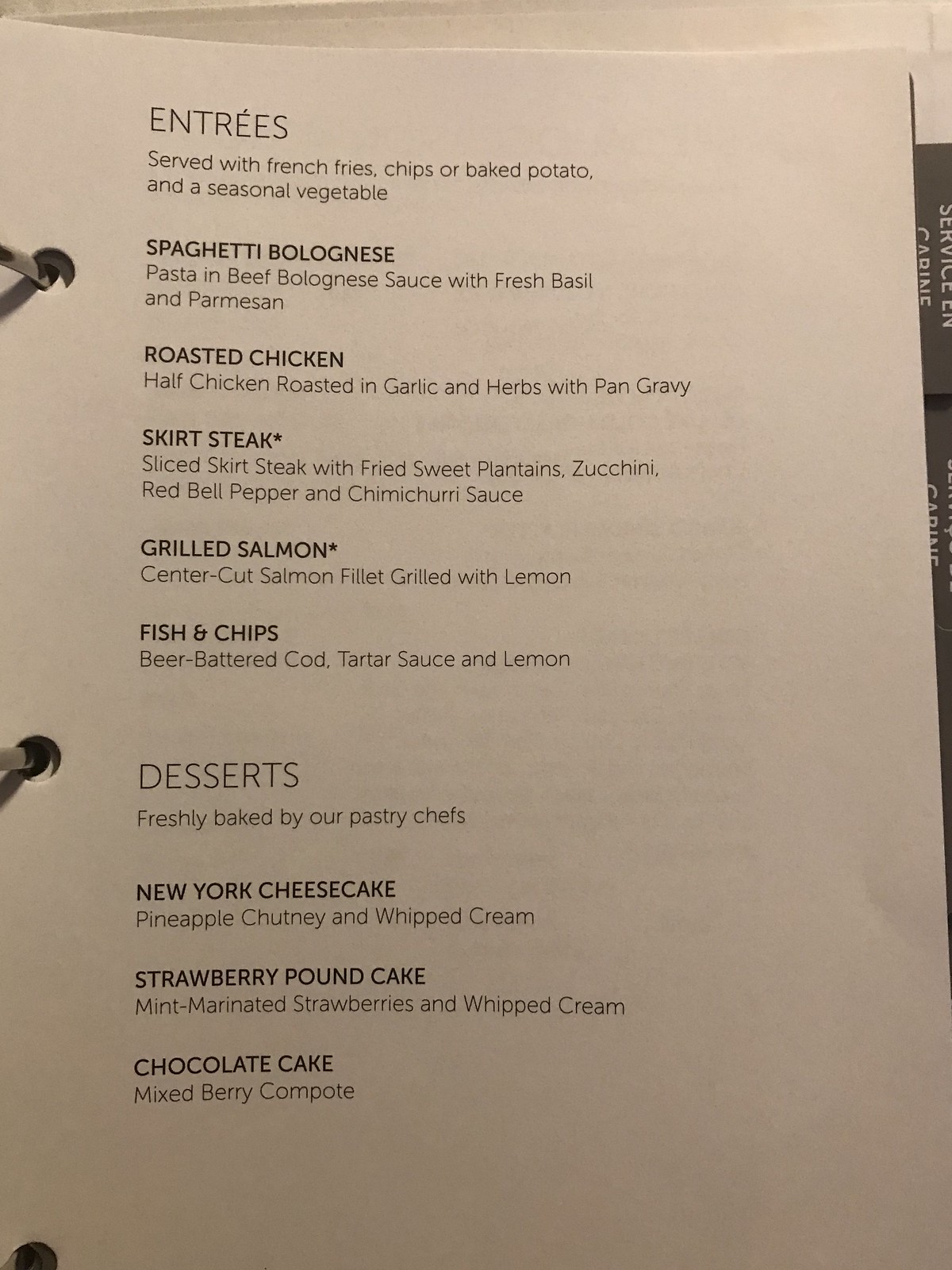A photograph captures an extensive restaurant menu, suggesting a comprehensive range of offerings. The menu is presented on thick white paper that resembles pages from a notebook, complete with tabs for easy navigation through its various sections. The background is stark white, providing no additional context about its surroundings or the surface it rests upon.

On the right edge of the menu, two black tabs are visible, though only one is partially legible, reading "service incarnate." The detailed list of offerings is printed in black ink and includes a variety of entrees and desserts.

**Entrees**:
- **Spaghetti Bolognese**: Pasta accompanied by a rich beef Bolognese sauce, garnished with fresh basil and Parmesan cheese.
- **Roasted Chicken**: Half a chicken, roasted with garlic and herbs, served with pan gravy.
- **Skirt Steak**: Sliced skirt steak paired with fried sweet plantains, zucchini, red bell pepper, and chimichurri sauce.
- **Grilled Salmon**: A center-cut salmon filet, grilled and served with a touch of lemon.
- **Fish and Chips**: Beer-battered cod served with tartar sauce and a slice of lemon.

The entrees come with a choice of french fries, chips, or a baked potato, accompanied by a seasonal vegetable.

**Desserts**:
- **New York Cheesecake**: Topped with pineapple chutney and whipped cream.
- **Strawberry Pound Cake**: Served with mint-marinated strawberries and a dollop of whipped cream.
- **Chocolate Cake**: Accompanied by a mixed berry compote.

Each dessert is freshly baked by the restaurant's pastry chefs, promising a delightful end to any meal.